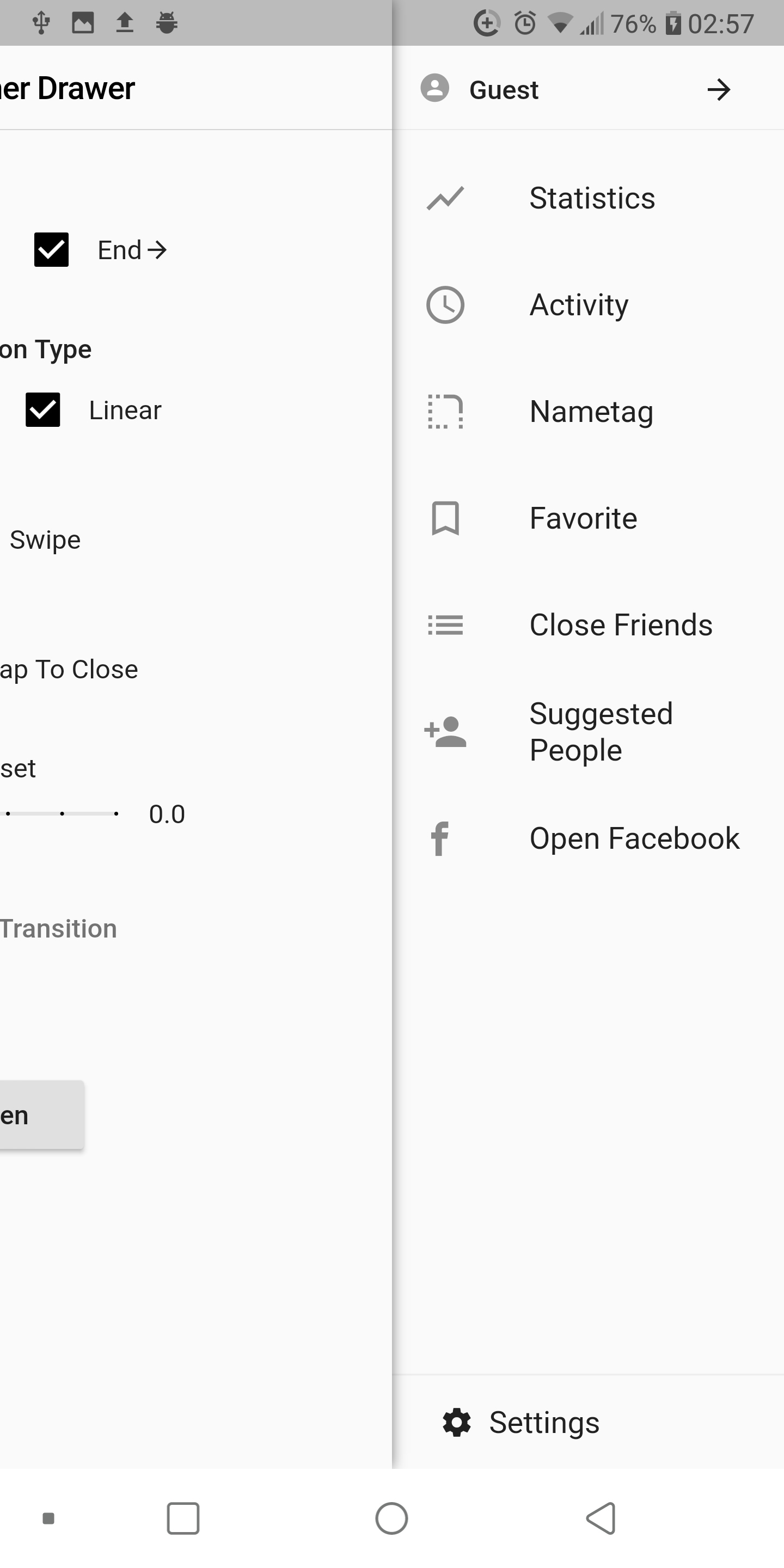Image Description:

The image features a white background and a drawer that extends from the right side. There's a highlighted checkbox that is checked and a line that ends with a right arrow. Another checked checkbox is partially visible, with the associated text cut off, possibly ending in "on." 

Below this, there is an entry labeled "linear" and the phrase "white think tap to close," with "tap" being partly visible. Further down, there are options that appear to be for setting or resetting, connected by a line that ends with "0.0."

Additional features on the image include labels and controls such as "transition," "guest," and an arrow pointing to the right. There are sections labeled "statistics," "activity," "name tag," "favorite close friends," and "suggested people." The content also includes prompts to "open Facebook" and various settings features. 

At the bottom of the image, there are icons, including a small shaded square, a larger unshaded square, a circle, and a left arrow made up of a triangle. The settings icon is also prominently displayed at the bottom of the interface.